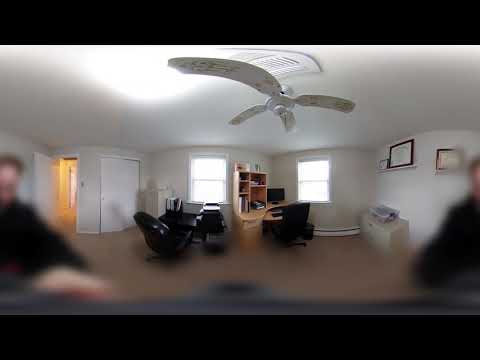In this blurry, likely fish-eyed or VR-distorted photograph, we are inside a room that appears to be a waiting area. The space is characterized by white ceilings and walls with a brown carpeted floor. A distorted ceiling fan is mounted above, barely discernible due to the heavy blur affecting much of the image. Along the back walls, framed certificates or diplomas suggest that this could be a professional setting, such as a doctor's or psychologist's office. There are two windows with sunlight streaming through, contributing to the overall brightness of the room. Chairs line the area near the windows, though they remain unoccupied. A door on the left side appears open, possibly leading to another room where indistinct figures of people can be seen waiting. Additionally, a cabinet is vaguely visible in the background. The photo's edges are particularly blurred, perhaps intentionally, for privacy or anonymity.